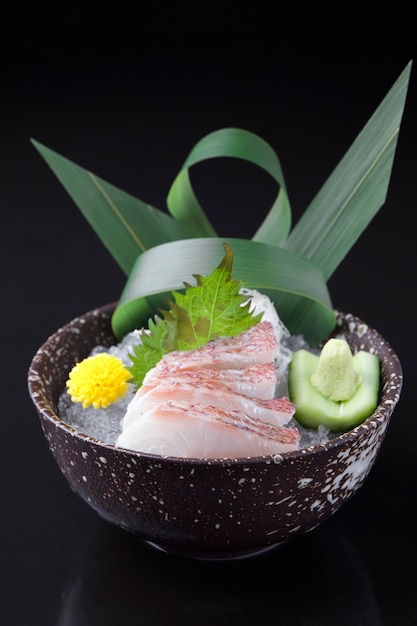In the photograph, a dark brown bowl with white speckles sits centrally against a completely black background, reflecting slightly on the surface below. Inside this speckled bowl, there are several slices of light pink fish, almost white on the sides, arranged neatly. Garnishing the fish is a small yellow flower with an attached green leaf leaning against it. Beneath the flower seems to be a base of crunched-up light gray ice. 

On the right side of the bowl, there is a chopped piece of vegetable, possibly celery, topped with a small yellow segment, suggesting a fruit or vegetable core. Behind this arrangement, a large green leaf is artistically shaped into cylindrical forms, one part pointing left and another right, adding a dynamic visual element. The fish appears seasoned with light black specks. The photograph, evidently taken indoors, captures meticulously arranged sashimi with a green twisty vine-like ribbon adding a playful touch behind the main items.